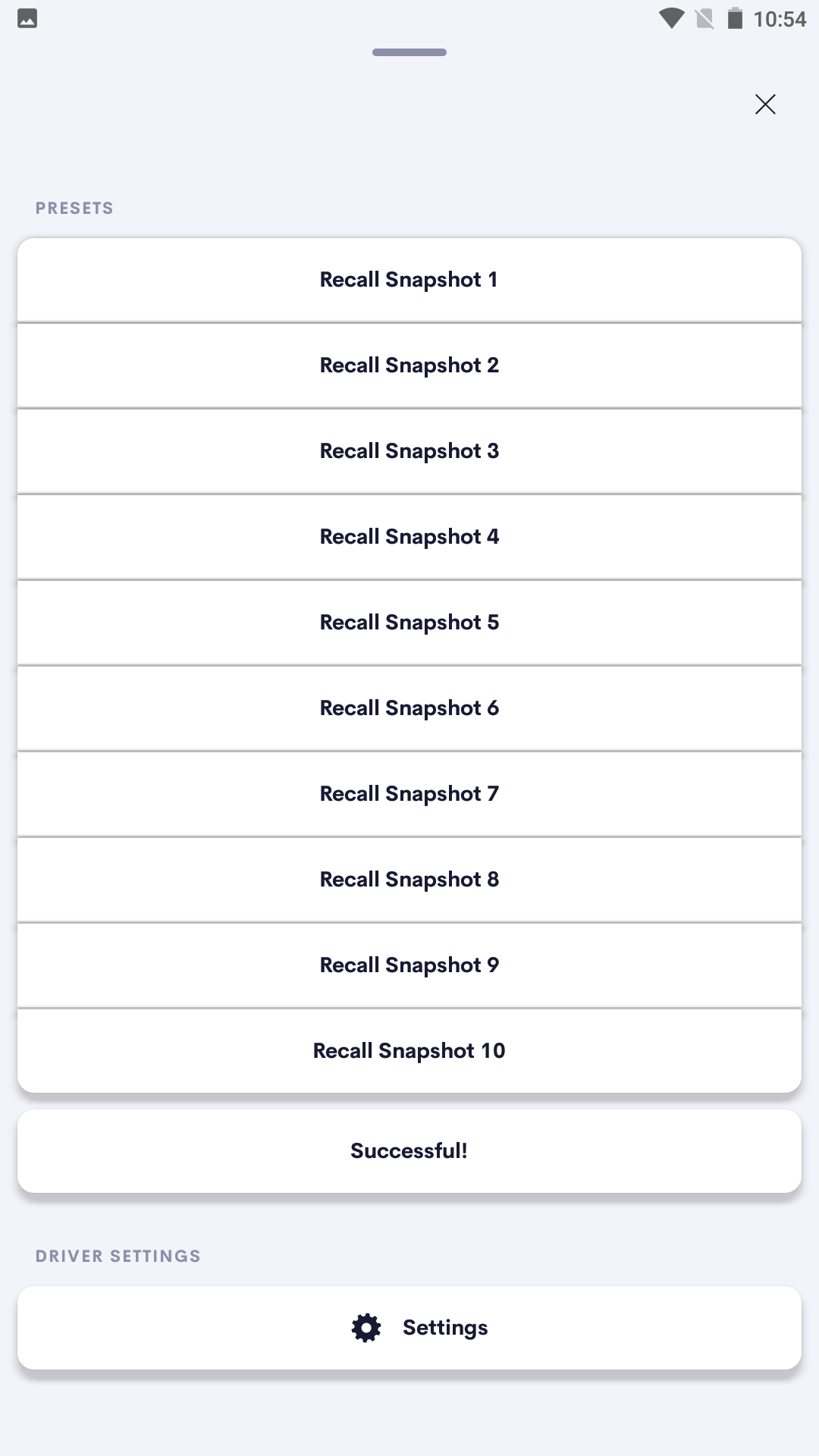This image is a screenshot from an image capture application, possibly associated with a specific smartphone brand. The screenshot prominently displays various functions and settings within the app. 

At the center of the image, there are presets labeled "Recall Snapshot 1" through "Recall Snapshot 10," indicating that the user has the option to quickly retrieve up to ten preset snapshots. At the bottom of these presets, a message states "Successful!" with an exclamation mark, suggesting successful recall or saving of a snapshot. 

An 'X' button located in the far right corner allows the menu to be closed. Below this, there are additional options labeled "driver settings" along with a gear icon that presumably opens the main settings menu. These menus are slightly elevated with subtle shadows underneath, and the text appears mostly in bold, lowercase letters with a touch of gray color. 

In the upper left corner of the image, an icon resembling a photo app — a small square with a mountain silhouette against a dark background — further suggests this app’s association with image management or recall. 

Other screen details include the status of the phone: the Wi-Fi is turned off, as indicated by the black Wi-Fi icon, the battery is nearly full, and the current time is displayed as 10:54, though it's unclear whether it's AM or PM.